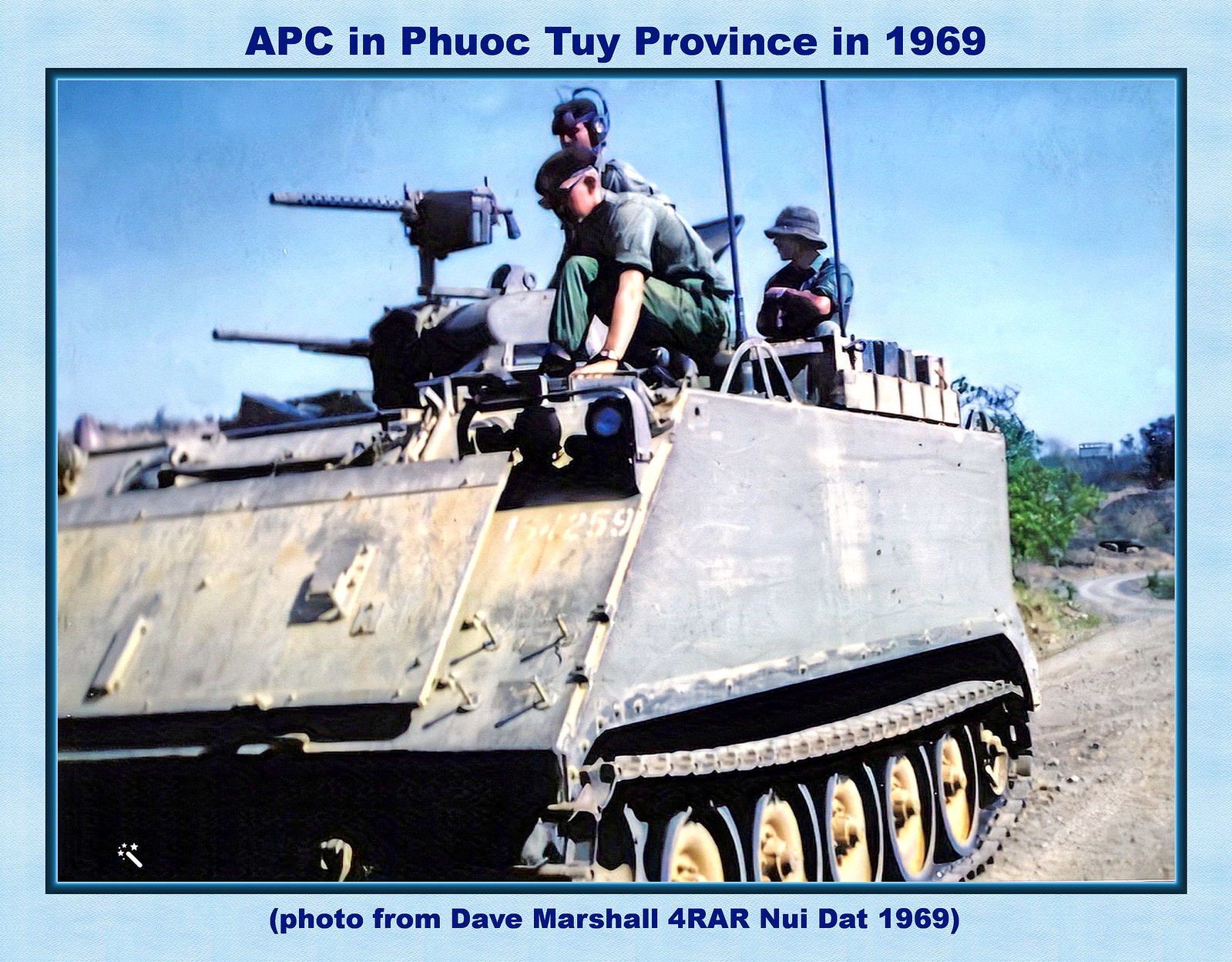In a historical photograph from 1969 titled "APC in Phuoc Tuy Province," set against a powder blue background with a dark blue border, a large, silver-gray military tank dominates the scene. This armored vehicle features two projecting scopes, one resembling a gun barrel, as well as two front lights—one illuminated in blue and the other unlit. Yellowish wheels support the tank, which rests on a dirt road stretching back into a landscape of green foliage under a clear blue sky. Atop the tank, three men are perched: the rear man wears a fisherman's hat, the middle man dons an unclear apparatus perhaps for radio transmission, and the front man, hatless, sports glasses. The title and caption of the image identify its location as Phuoc Tuy Province, with a subtext crediting the photo to David Marshall for RAR Nui Dat 1969.